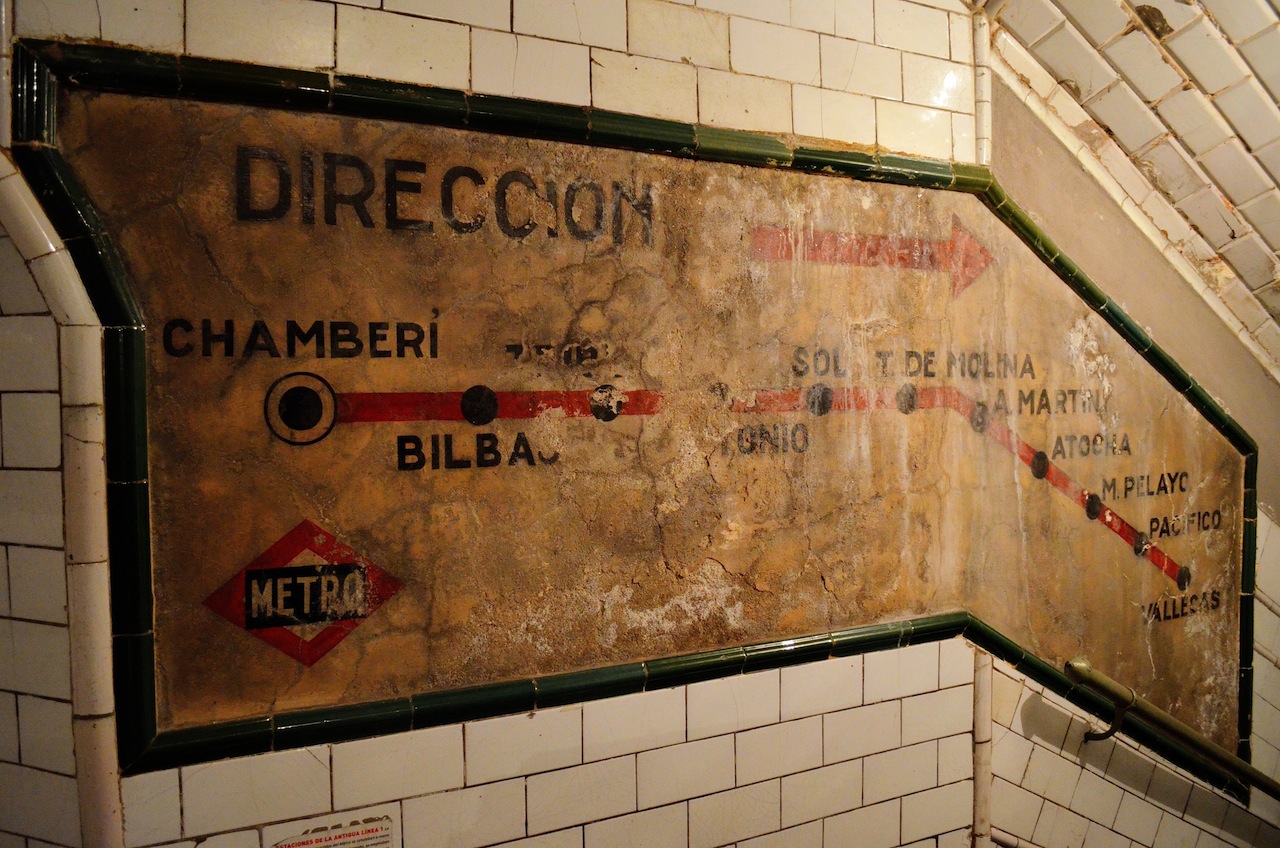This image captures a decrepit section of a metro station, its sign visibly worn and neglected. The sign bears the word "Metro" in the top corner and "Dirección" at the top, guiding commuters with arrows to the train platforms. The language suggests a Spanish-speaking country. The sign, illustrating the route with a red line adorned with black dots representing various stops, is incredibly old and faded, with many place names unreadable due to peeling and dirt. It is affixed to a wall of crumbling white tiles, partially surrounded by a green glass-tiled frame. The scene is brightly lit, casting shadows of a banister that indicates a nearby stairway leading down to the platform. Overall, the station is in desperate need of repair and cleaning, reflecting years of wear and tear.